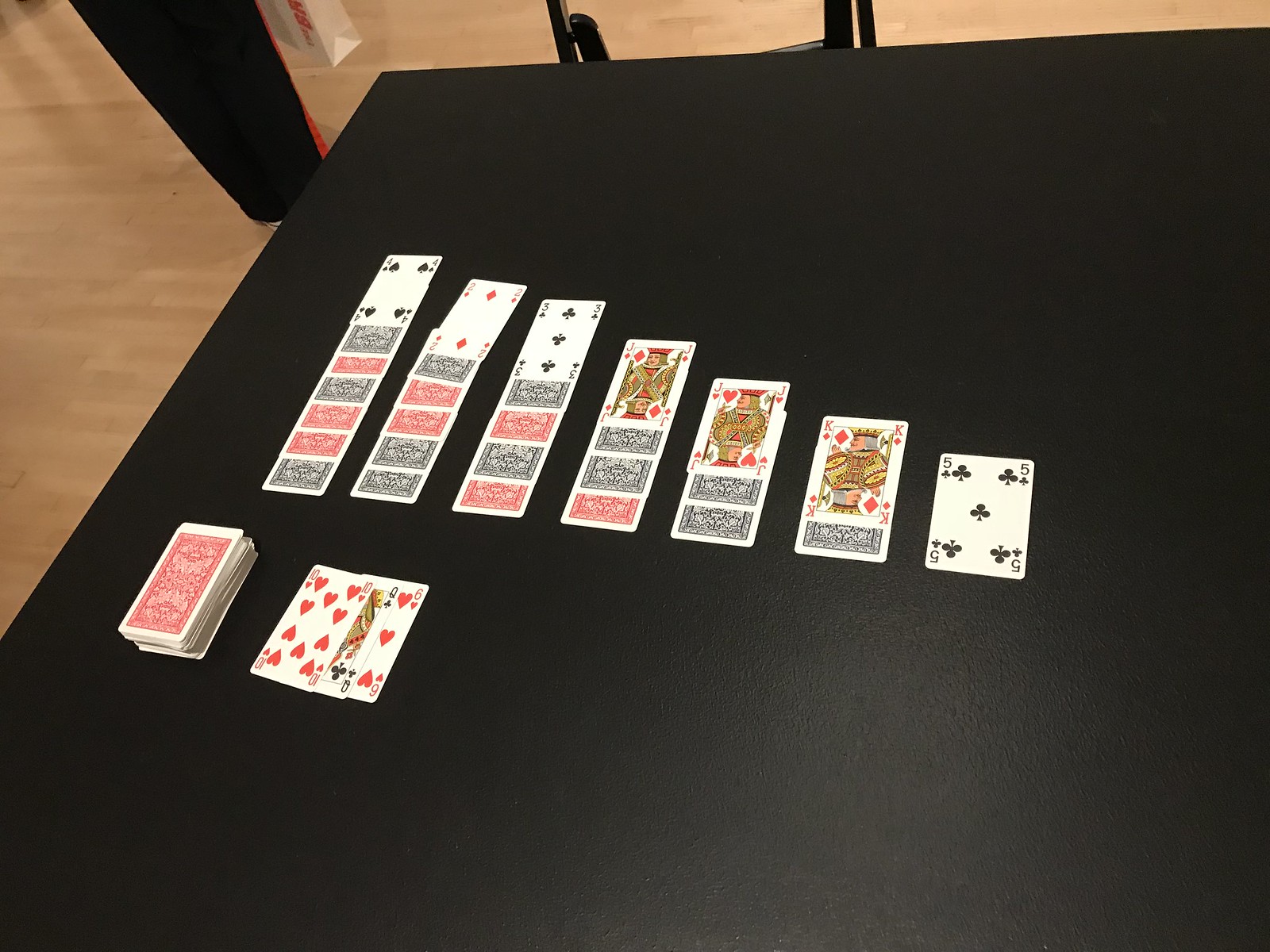In this image, a room with a light, elegant wooden floor sets a serene ambiance. In the center, a tall figure, possibly a person dressed in black with red accents, stands beside a white bag that has specks of red on it. To the side, a black metal chair is partially visible. Dominating the scene is a large table draped with a black cloth. Atop the table, a deck of cards lies spread out. The deck, with red backs and white edges, has its majority face down. Nearby, three cards are face-up, indicating an ongoing game of solitaire. The solitaire setup includes seven rows of cards. The first row has one card turned up, the second row has one card up and one down, and the pattern continues to the seventh row, which has six cards down and one card up. The backs of the cards vary in color, with some being blue and others red, creating a striking contrast on the table.